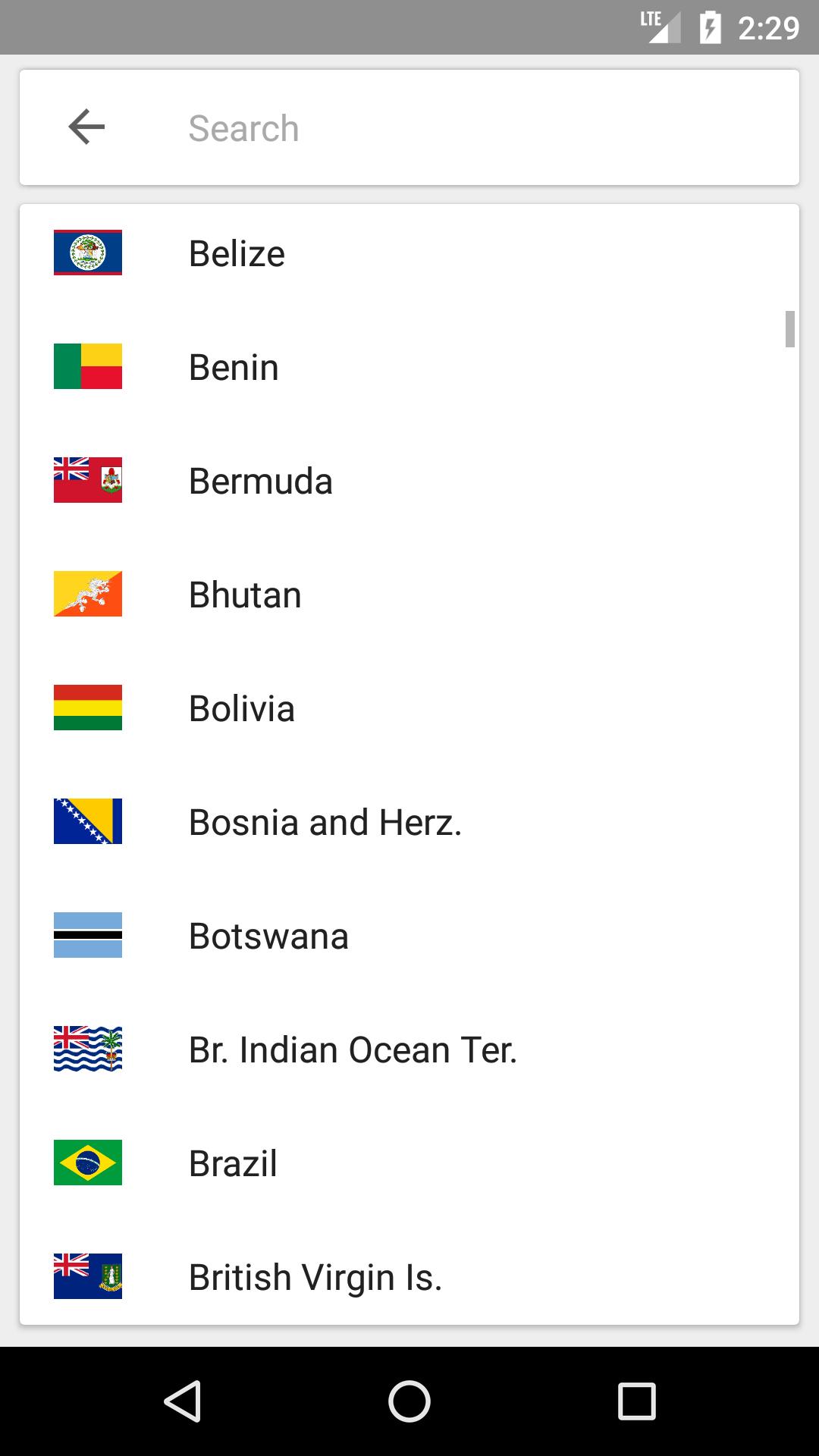Here is a polished and detailed caption based on your description:

---

This image captures a smartphone screen displaying an application interface. At the very top of the screen, there is a gray status bar featuring a white LTE service indicator, battery icon, and the current time, "2:29". Below the status bar, there are two large boxes with white backgrounds encased in light gray borders. 

The top box is thin and contains a placeholder text "Search" in gray, accompanied by a black back arrow on the left side. Below this is a larger box with a scroll icon on its right. This section lists countries along with their respective flags, arranged alphabetically. The countries, displayed in black text, include Belize, Benin, Bermuda, Bhutan, Bolivia, Bosnia and Herzegovina, Botswana, British Indian Ocean Territories, Brazil, and British Virgin Islands. Each country’s name is paired with its colorful flag, which lacks any bordering. 

At the bottom of the screen, a black navigation bar houses three white outline icons: a back arrow on the left, a circle in the center, and a square on the right. The centers of these icons are transparent, revealing the black background. 

Overall, the image depicts a neatly organized list of countries within a mobile application, highlighting its simple and efficient user interface.

---